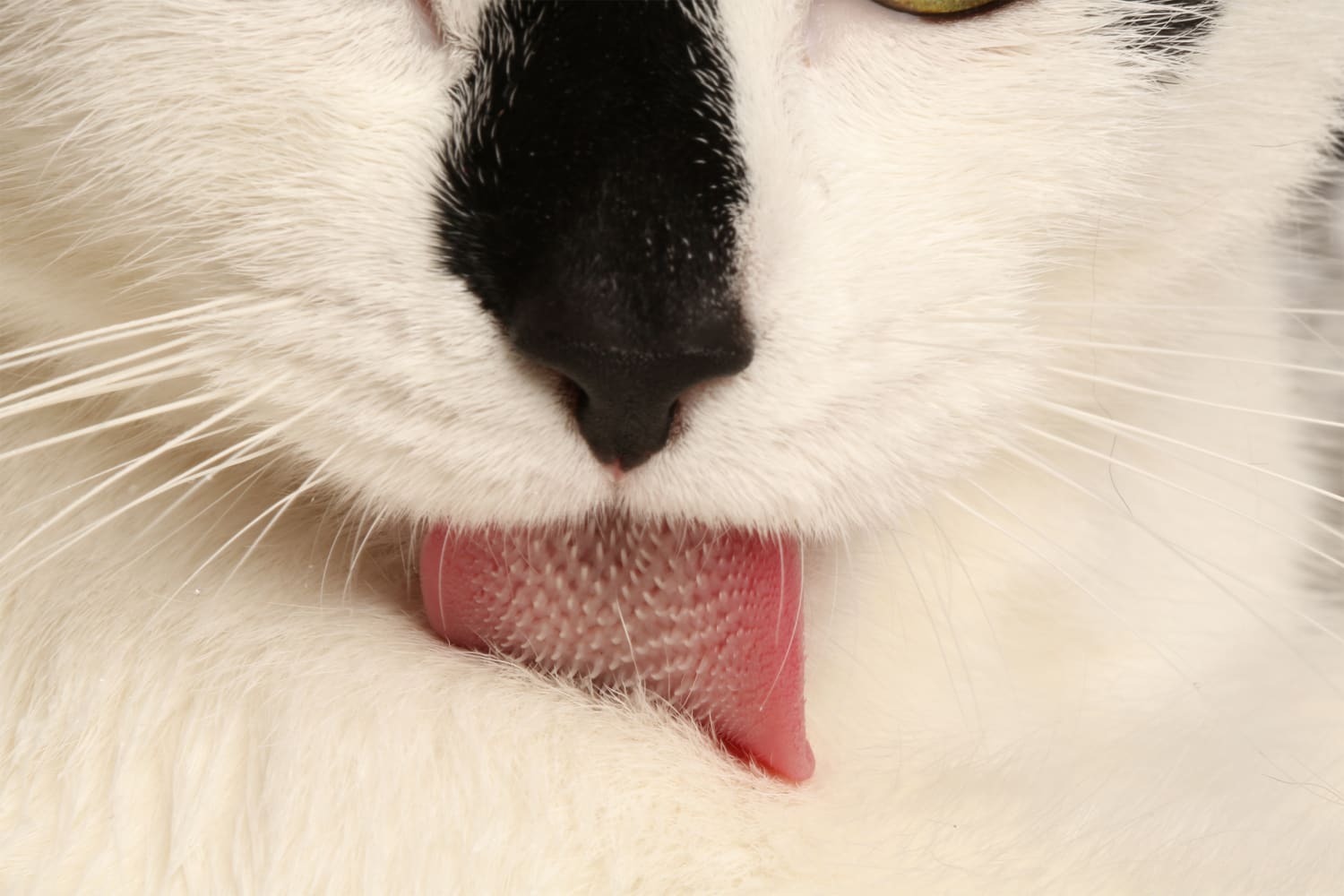This is an extreme close-up photograph of a cat's face, zoomed in to the point where the eyes are almost entirely cropped out, revealing just the bottom edge of the right eyelid. The cat has striking white fur and prominent white whiskers that fan out around its face. The center of the image features its bold black nose, surrounded by short black fur that extends slightly above it. The cat is engaging in a grooming activity, sticking out its bright reddish-pink tongue to lick its own fur. The incredible zoom level of the photo allows us to see the bristly texture of the tongue, which is adorned with tiny white, spiky protrusions used for cleaning. This intimate view captures the intricate details of the cat's grooming habits and facial features with remarkable clarity.